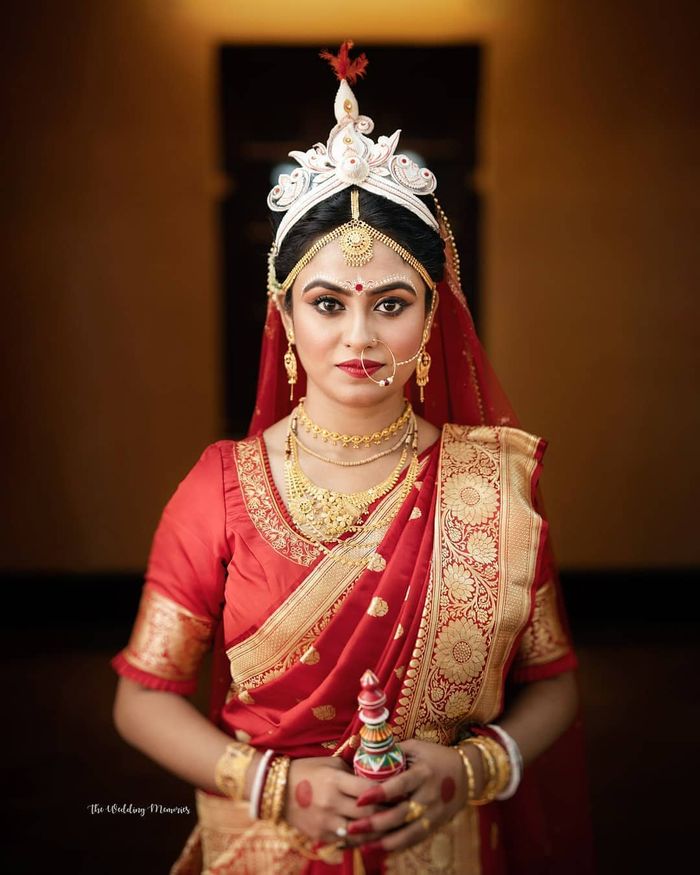The photograph, taken indoors against a blurred beige or orange wall, captures a woman adorned in traditional Indian wedding attire. She stands elegantly, posing in a vibrant red and gold sari, which features intricate gold floral patterns throughout. Complementing her elaborate outfit, she wears an ornate headdress with floral designs and dangling gold chains. Her forehead is decorated with a prominent red bindi, and she sports a large nose ring connected by a chain to her headdress. In her hand, she holds a pointed, ornate object. Her hands are adorned with red fingertips and numerous gold rings. She also wears multiple gold necklaces, bracelets, and other face jewelry. At the bottom of the image, partially obstructed white text reads "THE..." among other unclear words.